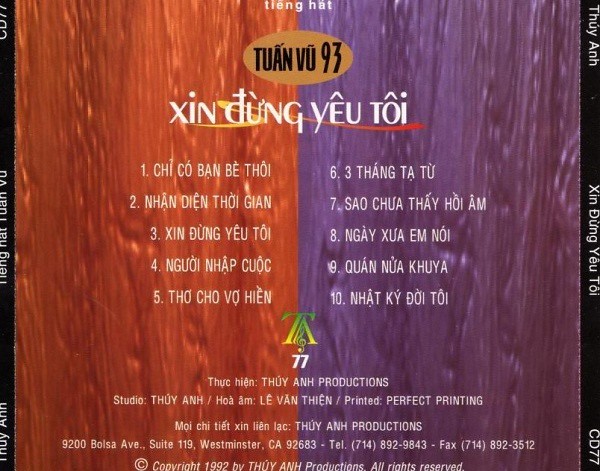This image is the back cover of a CD jewel case featuring a design divided into two distinct halves. The left half of the cover boasts a red, oily-textured background, while the right half features a purple, similarly textured background. This split design accentuates the tracklist, which is numbered from 1 to 5 on the red side and from 6 to 10 on the purple side. At the top, "T-U-A-N-V-U-9-3" is prominently displayed, followed by the title "Zing Yeutoi" (spelled Z-I-N-G Y-O-U-Y in English). Below this is a green T-N-A and the label A-N-H Productions. In the bottom right corner, "CD 77" is inscribed along with the first track named "Chico Band-Aid Toy". The bottom of the cover declares, "Copyright 1992 by Thuy Anh Productions, all rights reserved." Surrounding this information, the edges are designed to fold and secure the CD tray within the jewel case. The majority of the text is in Vietnamese, indicating the origin and content of the CD, which includes a complete list of ten songs.